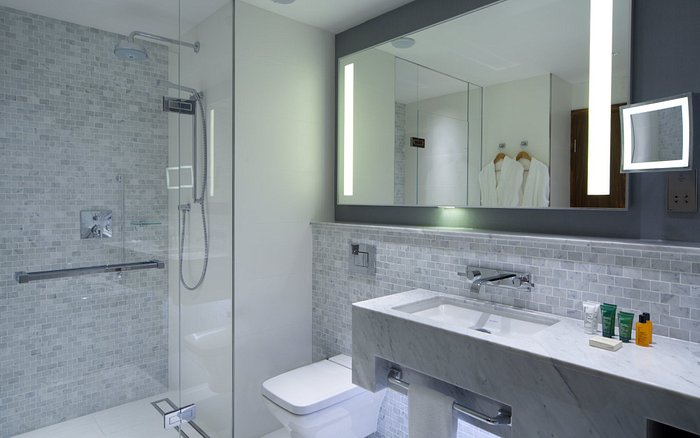The image depicts the interior of a modern bathroom, exhibiting sleek architectural design and contemporary styling. To the left side of the room is an upright shower unit with transparent glass doors and a non-detachable shower head positioned at the top. The surrounding walls are adorned with light gray square tiles, contributing to a unified aesthetic as this tiling extends into the shower area as well.

To the right side, there is a stylish floating vanity made of light gray and white marble. Despite featuring two sinks, only one square sink is visible in the image. Above the vanity, a large rectangular mirror spans the wall, flanked by two vertical, rectangular light panels that provide a warm ambiance. The reflection in the mirror reveals a cabinet and additional details of the shower system, along with two white robes hanging neatly on wooden hangers.

Below the mirror and to the right, there is an assortment of toiletries including lotions, bottles, and a bar of soap neatly arranged on the countertop. Adjacent to the vanity, and to the left, a sleek, modern white toilet without an attached tank enhances the minimalist aesthetic of the space.

At the bottom center of the image, towels are hanging, suggesting easy access and convenience for the user. The lighting within the room is modern, featuring a square light fixture that complements the overall contemporary design theme.